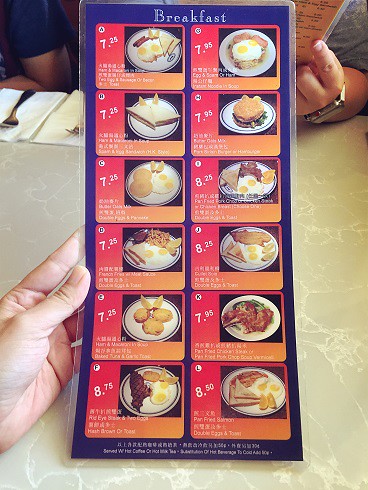A left hand holds up a plastic-covered breakfast menu, prominently framed by a dark blue border at the top with bold white text announcing "Breakfast." The menu is divided into twelve squares, arranged in two columns of six, each showcasing different breakfast dishes. The dishes, such as bacon and eggs, eggs and toast, and sausage, are all presented on white plates. Each square is visually distinct with a red background at the top and an orange background at the bottom. Next to the images of the dishes, prices are displayed in white text, ranging from $7.25 to $8.75. Below each image, there is additional white text providing some description, although it is not legible. The light greenish marble surface of the table in the background adds a sophisticated touch to the scene. Another individual is partially visible in the background, their hand also holding a menu, suggesting they are similarly engrossed in breakfast selections.